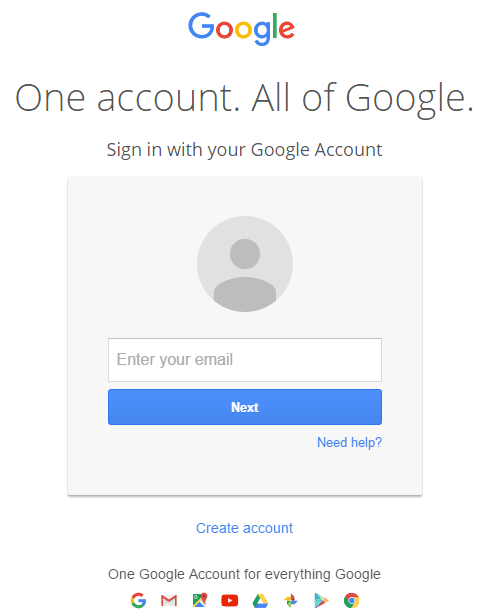The image showcases the sign-in page for Google on a mobile phone. Dominating the top center is the iconic Google logo. Beneath it, the text reads "One account. All of Google." In smaller print below, it instructs users to "Sign in with your Google account."

A white input field is situated below, adorned with a light gray circle displaying a simple person icon— a circular head above a curved line representing the body. This field prompts users to "Enter your email." Directly underneath, a blue button labeled "Next" is visible. To the right of this button, there is a "Need help?" text link with a question mark.

The entire white panel has a subtle drop shadow, giving it a slight elevation effect. At the bottom of this panel, there is an option to "Create account," followed by a reassurance that "One Google account for everything Google" can be created.

At the very bottom of the screen, eight icons are lined up: the letter 'G' for Google, the Gmail envelope, the Google Maps pin, the YouTube play button, an icon possibly representing Google Drive or Google Cloud, a database-like icon, a pinwheel icon, a right-facing triangle for the Google Play Store, and finally, the circular logo for Google Chrome.